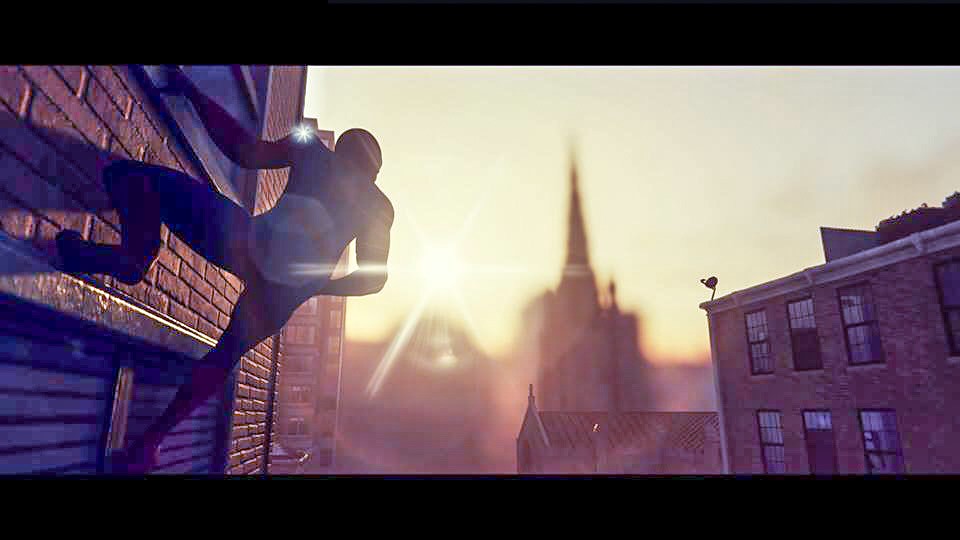This detailed screen capture, likely from an animated film or video game such as "Spider-Man" on the PS4 or PS5, features Spider-Man in his iconic suit clinging to the side of a reddish-brown brick building on the left side of the frame. Spider-Man's pose is dynamic: his right leg is bent and propped above what appears to be a door, while his right arm grasps a windowsill. His left leg stretches downward, foot planted on a bluish, horizontally lined surface that could be a shaded window, and his left arm rests near his waist. A brilliant light from the setting or rising sun silhouettes Spider-Man, creating starbursts of light just above his right shoulder. The sunlight casts him almost entirely in silhouette, accentuating his pose against the bright backdrop.

To Spider-Man's left and towards the image's horizon, the city skyline is visible. The neighboring building, also made of brownish brick, features six fully visible windows, two of which are open, outlined in black with grating. This building includes decorative stone molding along the top and a small satellite dish at the left corner. In the distance, the blurred shapes of a church steeple and another possibly tiled-roof building can be seen. A billboard peeks from behind these structures, along with hints of trees and other urban features set against the sunlit sky. The bottom and top of the image are bordered by thin black bars, resonant of a widescreen movie format.